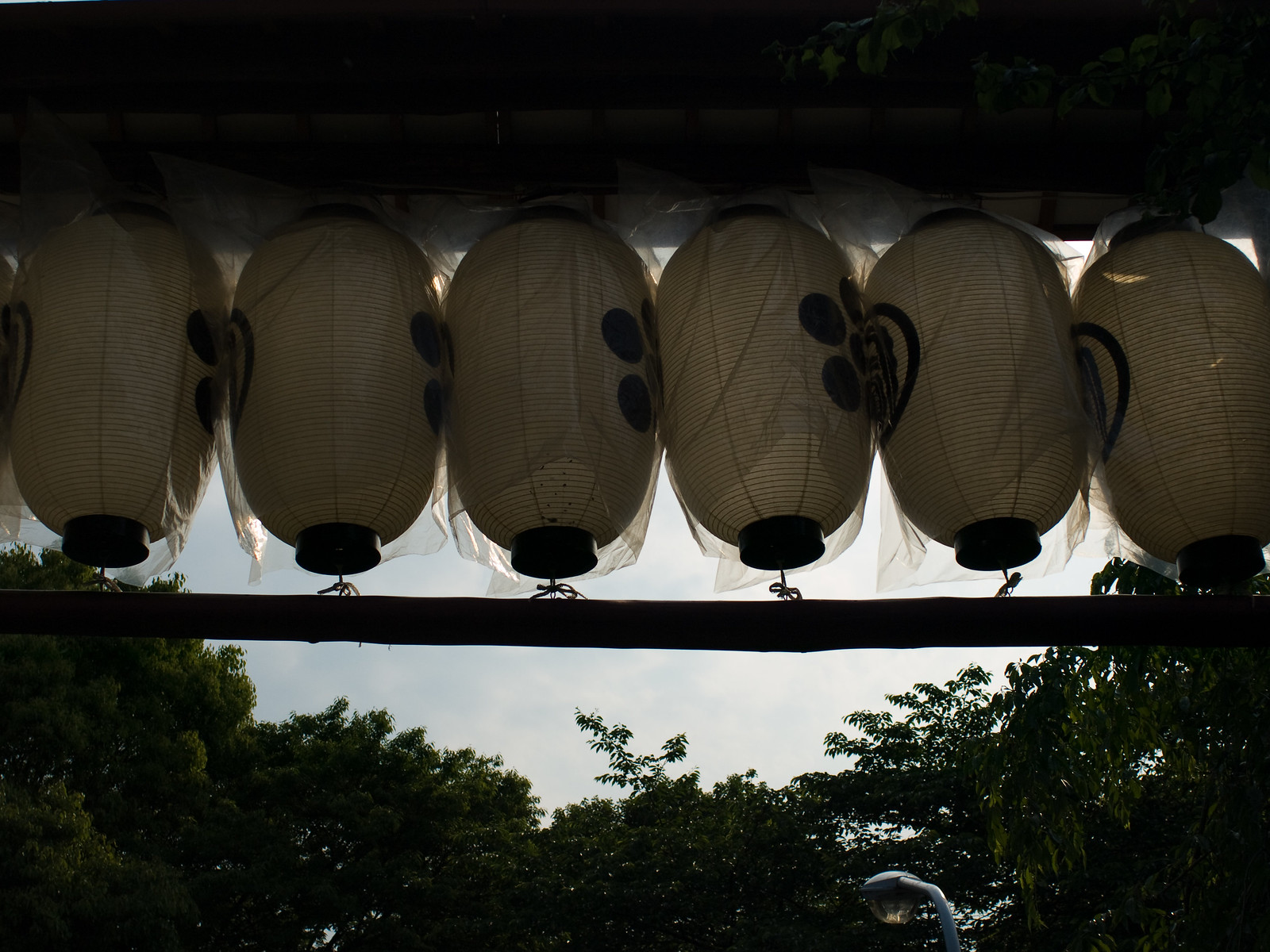This landscape-format photograph captures six Japanese-style paper lanterns hanging from a brown wooden rafter in an outdoor shed. Each white lantern features distinctive designs: four of them showcase a large black floral motif comprising circles on one side and an open black circle with a line on the other. The lanterns have black tops and bases and are still wrapped in plastic, indicating they have not yet been used. Below the lanterns, there is another brown wooden cross piece. The scene extends to an outdoor area with various green treetops against a grey, overcast sky. A silver street lamp with a white globe is visible, adding to the ambiance of the image.